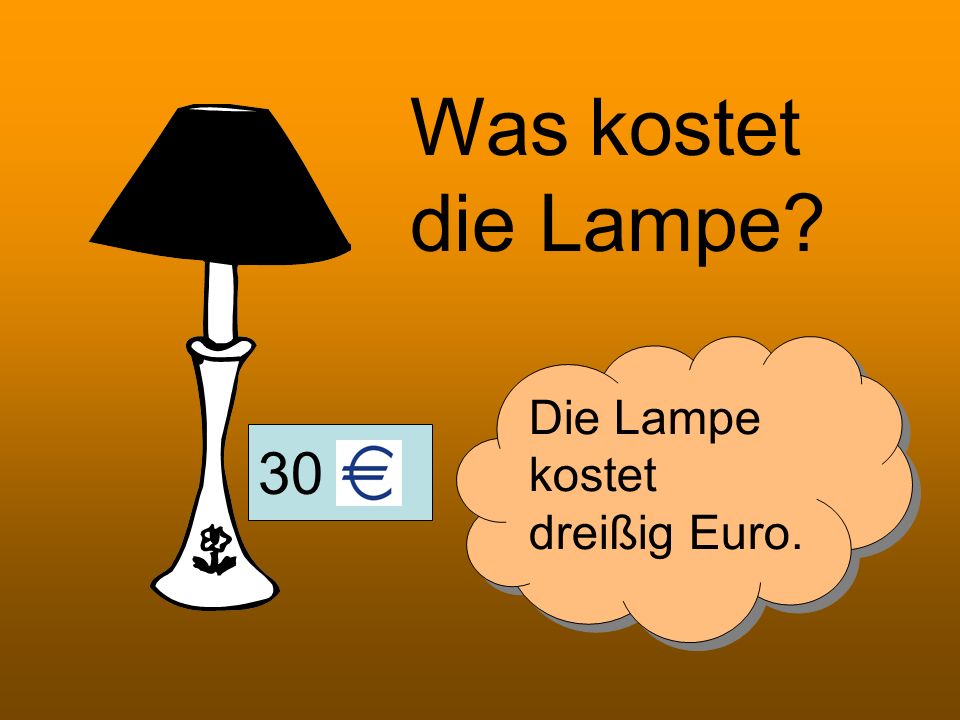The image features a distinct background that transitions from orange at the top to brown at the bottom. On the left side, there is a stylized, cartoon-like white lamp with a black flower design at its base and a black lampshade. In the center, a light blue rectangle contains the number "30" followed by a euro symbol, indicating a price of 30 euros. On the top right in black text, it reads "WAS KOSTET DIE LAMPE?" which translates to "How much is the lamp?" Beneath this, within a beige, cloud-like shape bordered in gray, is the repeated phrase "DIE LAMPE KOSTET DREIßIG EURO," meaning "The lamp costs thirty euros."